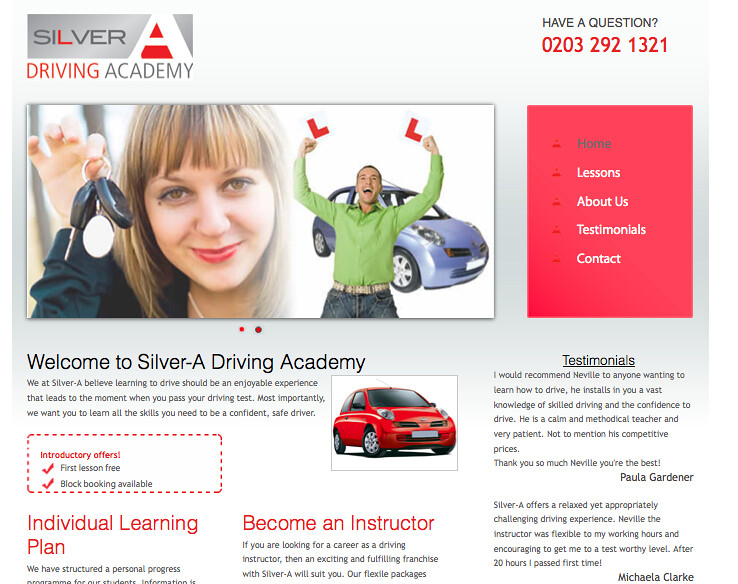The image is a screenshot of a website for Silver A Driving Academy. In the top left corner, there is the company’s branding and logo with "Silver" in gray text and the "L" in red, set against a gray background block with a stylized 'A' letter formed by a triangle cut in half. The top right corner features the text "Have a question?" followed by the phone number 0203-292-1321. The central part of the image prominently displays a welcoming headline, "Welcome to Silver A Driving Academy," and a tagline promoting an enjoyable and comprehensive learning experience leading up to passing the driving test and becoming a confident and safe driver.

Below this headline, there is a smiling young woman holding car keys accompanied by a photo of a man in a green dress shirt cheering with his fists in the air, standing in front of a blue car. To the right of these images is a navigation menu with options such as Home, Lessons, About Us, Testimonials, and Contact, set against a red background.

Further down, the image showcases introductory offers including a free first lesson and blog booking availability. There are sections with headings like "Individual Learning Plan" and "Become an Instructor." Additionally, the lower right part of the screenshot contains testimonials from satisfied clients Paula Gardner and Michaela Clark.